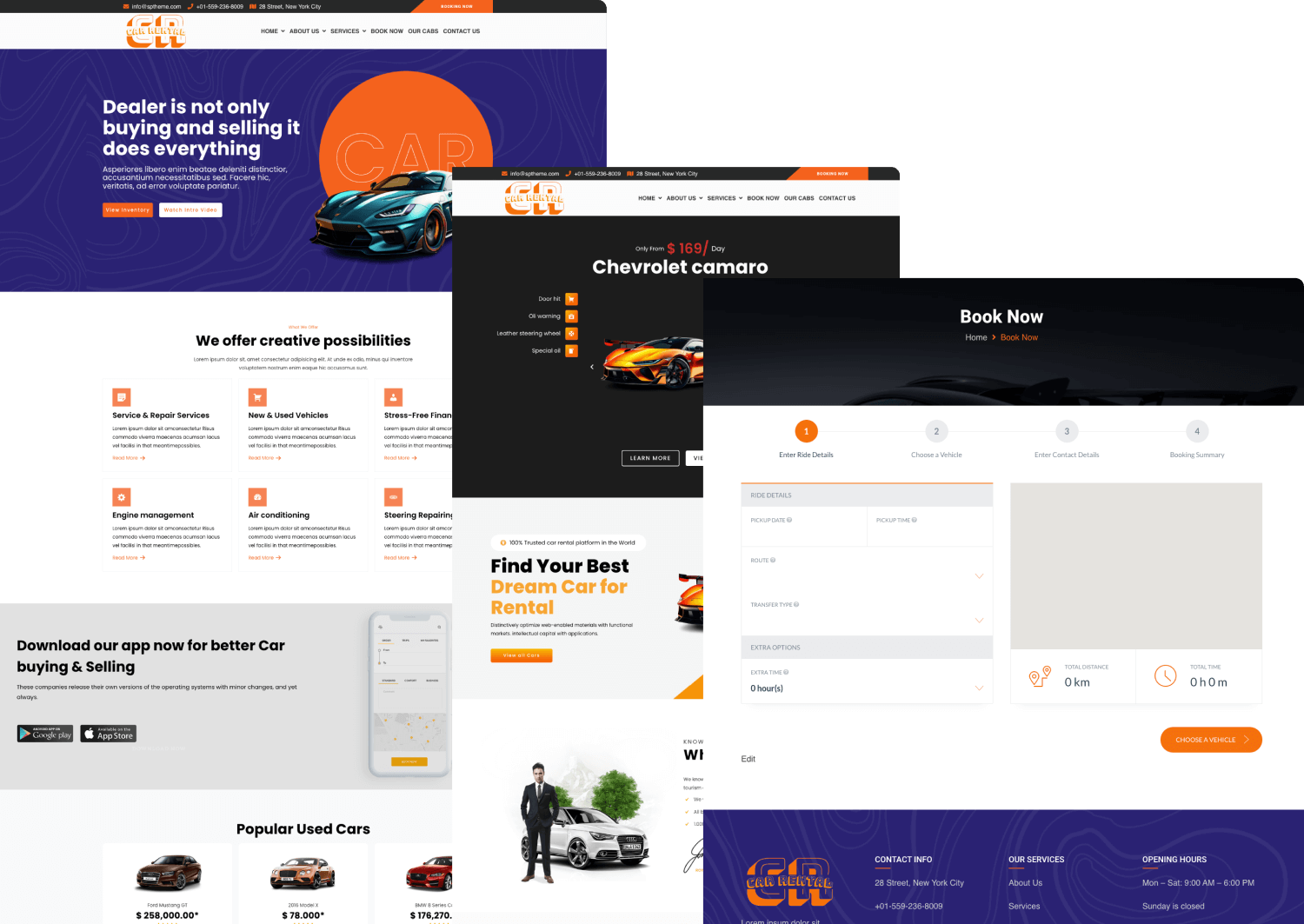Welcome to CR Bioservices, your comprehensive solution for all automotive needs. Our services encompass a vast range, from buying and selling vehicles to offering an extensive suite of repair services. As an MMPT-certified provider, our director oversees a varied inventory, including our standout orange rectangle speedster car. 

We provide stress-free engine management, air conditioning repairs, steering fixes, and more. Utilize our new app, available on Google Play and the App Store, for a seamless car buying and selling experience, complete with smart home integration. Whether you own a Chevrolet Camaro or another model, our platform allows you to easily book, manage, and track your vehicle's maintenance.

Visit us at 28th Street, New York City, or contact us at 015492368009. We are open Monday through Saturday from 9 am to 6 pm. Book your service today and experience the full spectrum of automotive care at CR Bioservices, where customer satisfaction and vehicle performance are our top priorities.